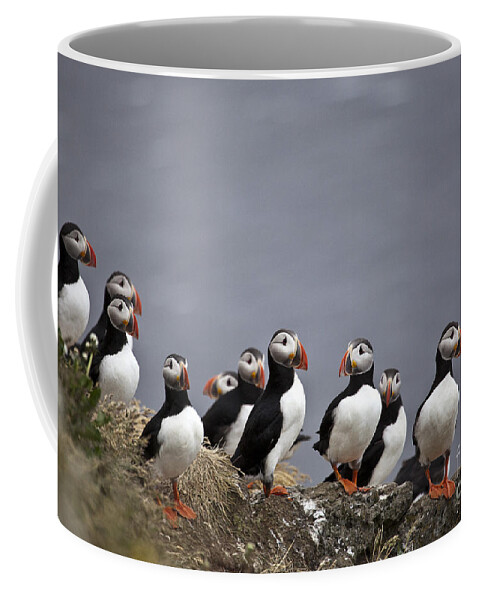The image depicts a standard white ceramic coffee mug, featuring a custom wrap-around design of puffins. These black and white birds, closely resembling penguins, are illustrated standing on a rocky and craggy ledge. The puffins, distinguished by their bright orange webbed feet and large triangular beaks, have white chests and faces with black heads, backs, and wings. They are depicted in various poses, facing different directions, against a backdrop of a murky, gray sky suggestive of impending snow. The mug’s inside is a creamy white, and the handle is of the same color. This whimsical and detailed scene of approximately ten puffins marching on an uneven ridgeline, amidst sparse wild bushes and grass tufts, encircles the entire mug, enhancing its charming uniqueness.